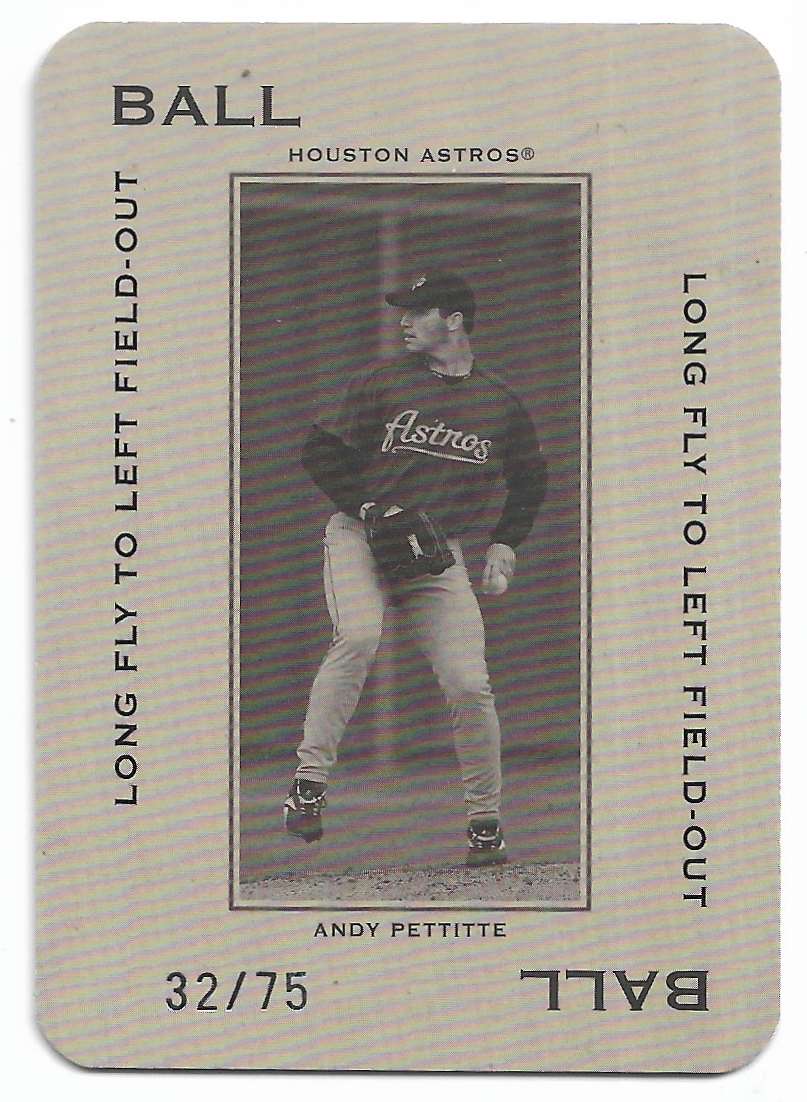This sepia-toned baseball card features Houston Astros player Andy Pettitte in a vintage style. The card captures Pettitte, dressed in an Astros jersey with a long-sleeve shirt underneath, black shoes, gray baseball pants, and a black Astros cap. He is pictured in a pitching stance, leg hiked up, ready to throw the ball with his left hand while wearing a mitt on his right. The phrases "LONG FLY TO LEFT FIELD OUT" are prominently displayed on both sides of the card. In the top left and bottom right corners, the word "ALL" repeats, with the bottom right instance appearing upside down. Pettitte’s name is spelled across the bottom in capital letters, and the card is numbered 32/75, indicating its limited edition status. The card also features a prismatic effect, giving it a distinctive, collectible sheen.